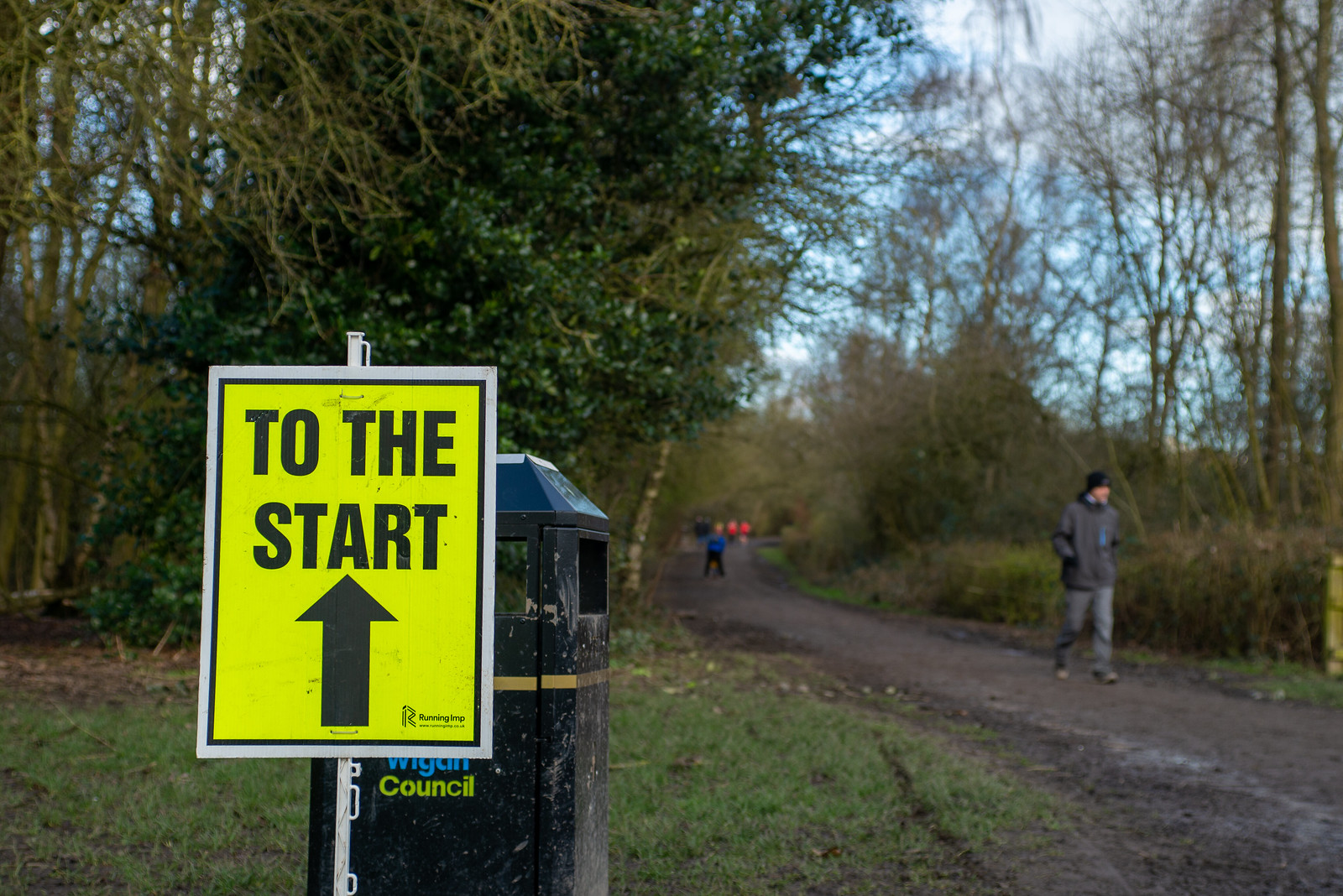The photograph captures a dirt walking path that winds through a wooded area. In the foreground, a man dressed in a gray sweatshirt, black ski cap, gray sweatpants, and blue jeans is seen walking alone on the path. To the left of the path, a prominent yellow sign with a white border stands out, reading "To the Start" in black font with a black arrow pointing upwards. The sign is mounted on a white metal pole anchored in sparse grass. Behind the sign, a black trash can bearing the words "Wigan Council" with "Wigan" in blue and "Council" in green, is visible. The surrounding wooded area consists of sparse, leafless trees and a few patches of green, indicative of recent rain making the ground appear dirty and muddy. The path extends far into the distance where several other people can be seen walking, framed by a sky dotted with white clouds and blue patches visible through the trees.